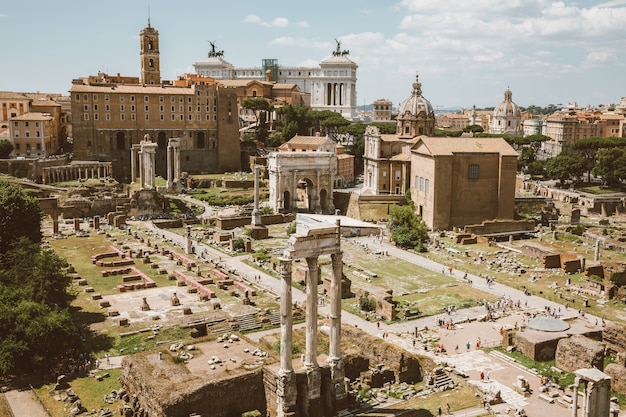The image captures an intriguing juxtaposition of ancient ruins amidst a developed urban landscape. At the center, there are remnants of an ancient civilization, including white pillars and stone foundations that suggest the former presence of grand, towering structures. These ruins, some featuring engraved letters, sit in a grassy area, possibly hinting at a former significant site, like a town square, city park, or even a cemetery.

Surrounding these historical fragments are multiple brown and orange buildings, displaying a mix of Victorian and European architectural styles. People stroll along the pathways weaving through the site, adding a dynamic, everyday touch to this scene of historical reverence. In the background, more modern, large apartment buildings loom, while closer to the ruins stand older, dome-shaped structures and steeples, all contributing to a sense of cultural progression over time.

A vivid blue sky with scattered white clouds crowns the scene, offering a serene backdrop to this complex blend of history and modernity. Notably, a small arc-like structure reminiscent of the Arc de Triomphe in France, though on a smaller scale, adds to the historical allure of this picturesque site.